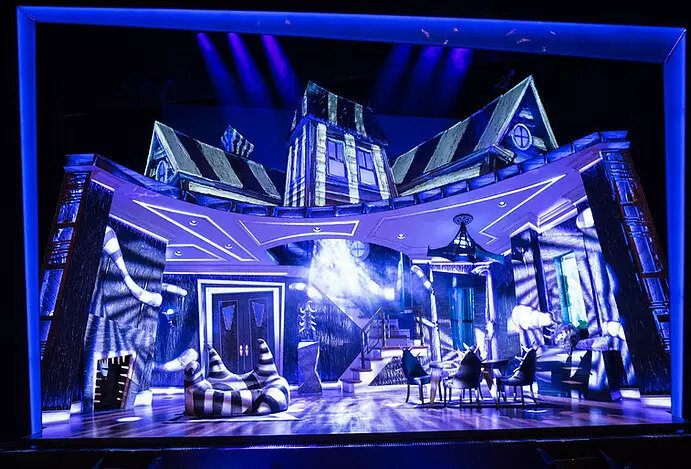The image appears to be a highly detailed, computer-generated scene of the interior of the Beetlejuice house, likely part of a stage set for a play or musical. The house is split open, allowing a view inside, which is illuminated primarily in shades of electric blue, purple, and accented with white and black. The room features a distinctive black and white striped couch that resembles Beetlejuice's iconic aesthetic, complete with witch-style points protruding from it. To the left, there's a whimsical fireplace adorned with teeth and a leg dangling down from it. In the right section, there's a dining table surrounded by chairs that have dagger-shaped protrusions. A sideboard with a bowl that has horns sits against the wall. A central winding staircase painted white leads to an upper level. The set also has peculiar, blob-shaped furniture, a light fixture hanging from the ceiling, a door towards the back of the room, and multiple roof sections striped in Beetlejuice's signature black and white pattern. The overall lighting creates a dark, eerie atmosphere, enhancing the fantastical and otherworldly feel of the scene.